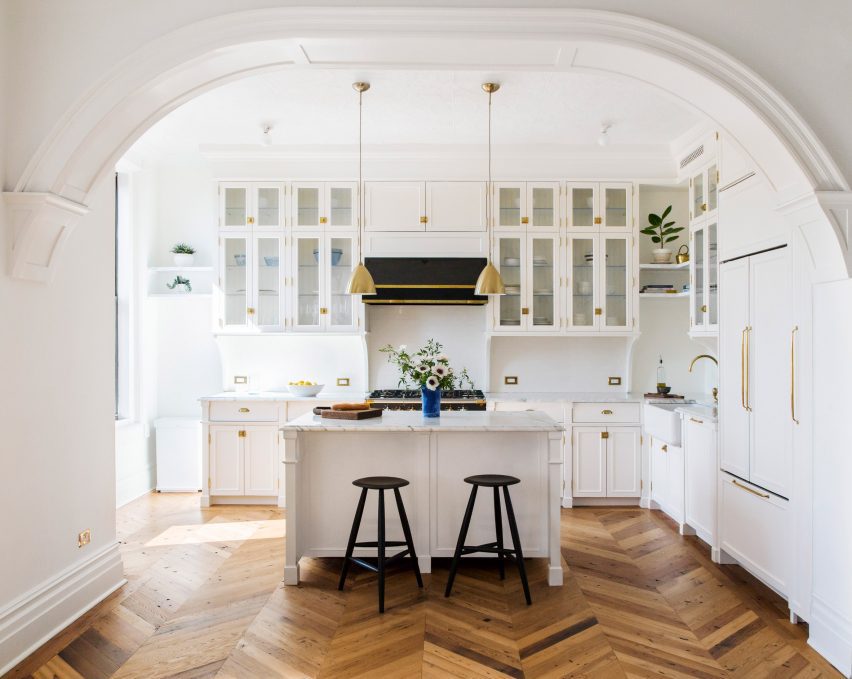This interior photograph showcases a bright and modern white kitchen with wooden herringbone floors displaying varying shades of natural wood. Dominating the center of the image is a pristine white kitchen island topped with elegant white marble. Atop the island sits a striking blue vase filled with white flowers, providing a splash of color. Flanking the island are two minimalist black stools made of wood. The kitchen is adorned with gold hardware throughout, with two gold-colored pendant lights hanging overhead. The white cabinets, complete with glass fronts on the upper sections, reveal neatly arranged dishes. A sleek white built-in refrigerator with gold handles blends seamlessly with the cabinetry. The background highlights a modern black stove hood above a black stove, contributing to the kitchen's sophisticated aesthetic. A subtle detail on the island includes a cutting board with a loaf of bread, further enhancing the lived-in charm of this contemporary space.